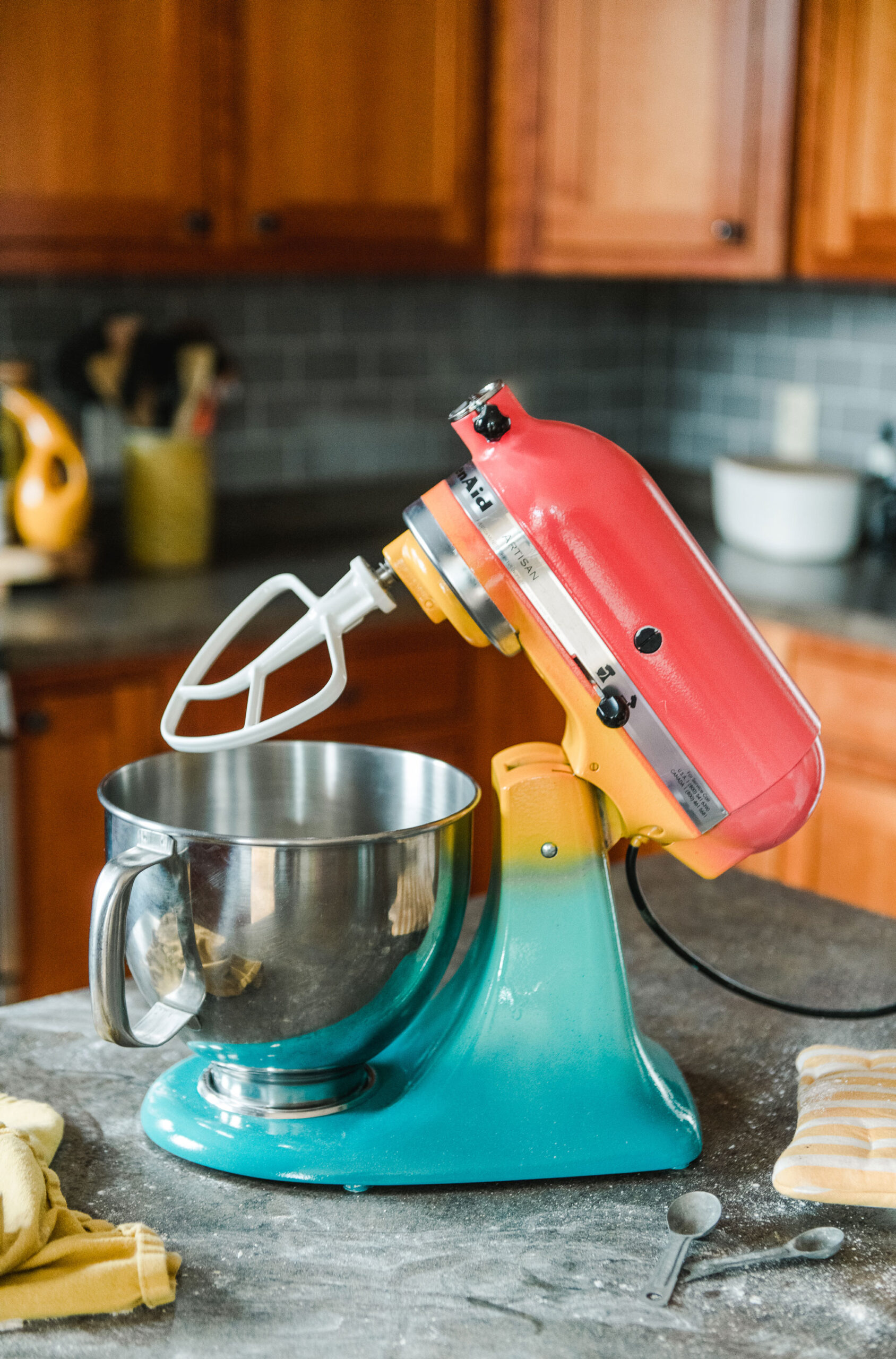In this clear and distinct photograph, a KitchenAid stand mixer takes center stage on a kitchen island. The mixer features a striking ombre design, transitioning from a blue base to yellow in the middle, and culminating in light red at the top. Its silver metal mixing bowl is equipped with an easy-grip handle, and a white dough attachment is prominently raised above the bowl, revealing the various components of the mixer. 

In the lower right of the image, two teaspoons rest on the counter amidst a light dusting of flour. Nearby, a blue or tan and white striped packet or cloth and a yellow cloth are also visible. The kitchen setting in the background, though blurred, showcases wooden cabinets, canisters, and a backsplash adorned with turquoise tiles. The countertops appear to be a grayish quartz and are adorned with various utensils, cookware, and a distinctive yellow bottle or decorative piece on the left side. The back room includes additional elements like black countertops and possibly more flour scattered around. The photograph captures both the stand mixer in detailed clarity and the inviting, somewhat busy atmosphere of a lived-in kitchen.